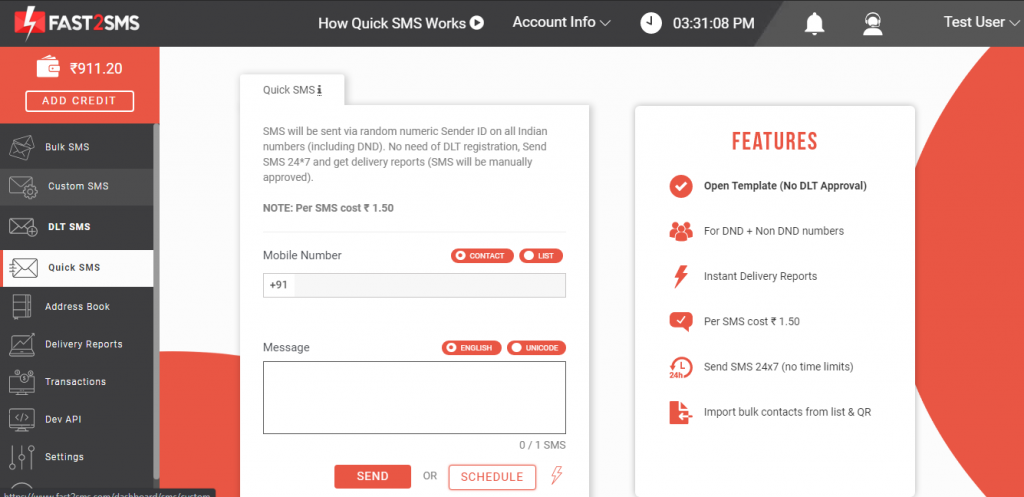This image is a screenshot of the Fast2SMS application interface, showcasing the various functionalities available to a user. The application icon, placed prominently in the top-left corner, features a red rectangle with a lightning bolt cutting through the middle. 

Along the left-hand side of the interface, there is a wallet icon displaying a balance of "911.20" units. Directly below this is a rectangular button labeled "Add Credit", allowing users to add funds to their account.

Following the wallet section is a list of various options associated with their respective icons. These include:
- Bulk SMS
- Custom SMS
- DLT SMS
- Quick SMS (highlighted with a white background to indicate it's the currently active option)
- Address Book
- Delivery Reports
- Transactions
- Dev API
- Settings

The central part of the screenshot is dedicated to the "Quick SMS" section, evident by a white background. This functional box features input fields for entering the recipient's mobile number and composing a message. Users have the option to either send the SMS immediately or schedule it for a later time. A note is clearly visible, stating that each SMS will incur a cost of "1.50" units.

On the right-hand side of the image is a "Features" box, detailing various features available for SMS options. 

The top portion of the interface is marked by a black or grayish bar, containing multiple action items. These include:
- An option to explore how Quick SMS works
- Account Information
- Current Date and Time

This detailed layout showcases both the user account management aspects and the core messaging functionalities offered by the Fast2SMS application.